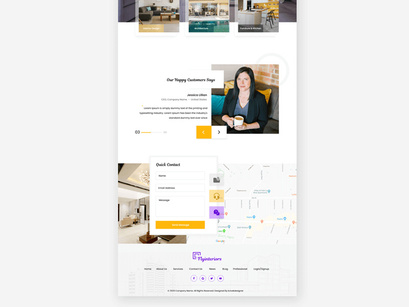The image is a low-quality screenshot, possibly from a real estate agency or housing website. At the top of the page, there are three images: one of a living room, a middle photo that is indiscernible, and the third appears to be of an office or kitchen island. Central to the page is a photo of a middle-aged woman, seemingly in her 40s. She is wearing a black blazer over a grayish tweed v-neck blouse and is holding a cup of coffee while looking directly at the camera with a smile. Her collarbone-length black hair frames her face as she sits on a couch against a brick wall with cushions. Adjacent to her picture is a caption that appears to begin with "Our happy customer" (possibly 'Kaya'), though the text is unclear. Below her image is a testimonial, but the content is too blurry to discern. The bottom of the page features a section labeled "Quick Contact", providing a space for visitors to get in touch with the page's administrator.